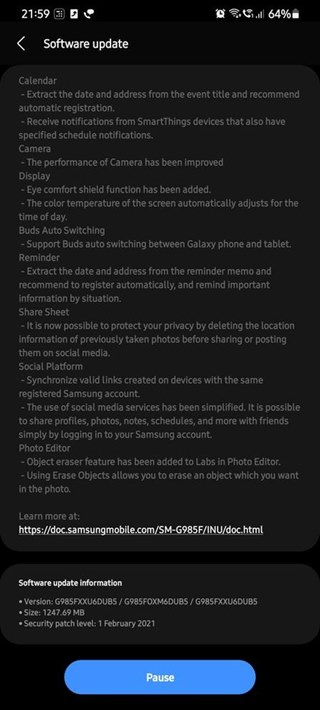**Caption:**

This detailed image of a Samsung mobile phone screen captures a software update notification at 21:59 (9:59 PM). The phone's battery is at 64%, and the Wi-Fi is connected. The user is currently on an active phone call while reviewing the update details. The notification highlights several new features and improvements:

- **Software Update Calendar**: Automatically extracts dates and addresses from event titles for automatic registration and receiving SmartThings device notifications with specified schedules.
- **Camera**: Enhanced performance.
- **Display**: Introduction of the Eye Comfort Shield, which adjusts the screen's color temperature based on the time of day.
- **Buds Auto Switching**: Supports seamless switching between Galaxy phone and tablet.
- **Reminder**: Automatically extracts and registers dates and addresses from reminders, ensuring important information is highlighted by context.
- **Share Sheet**: New privacy feature allowing deletion of location data from photos before sharing on social media.
- **Social Platform**: Simplified sharing of profiles, photos, notes, and schedules by logging into the Samsung account.
- **Photo Editor**: Addition of the "Object Eraser" feature in Labs, enabling users to remove unwanted objects from photos.

For further details, users are directed to a provided link. The notification also displays software version information, update size, security patch level, and features a blue 'Pause' button to temporarily stop the update process.